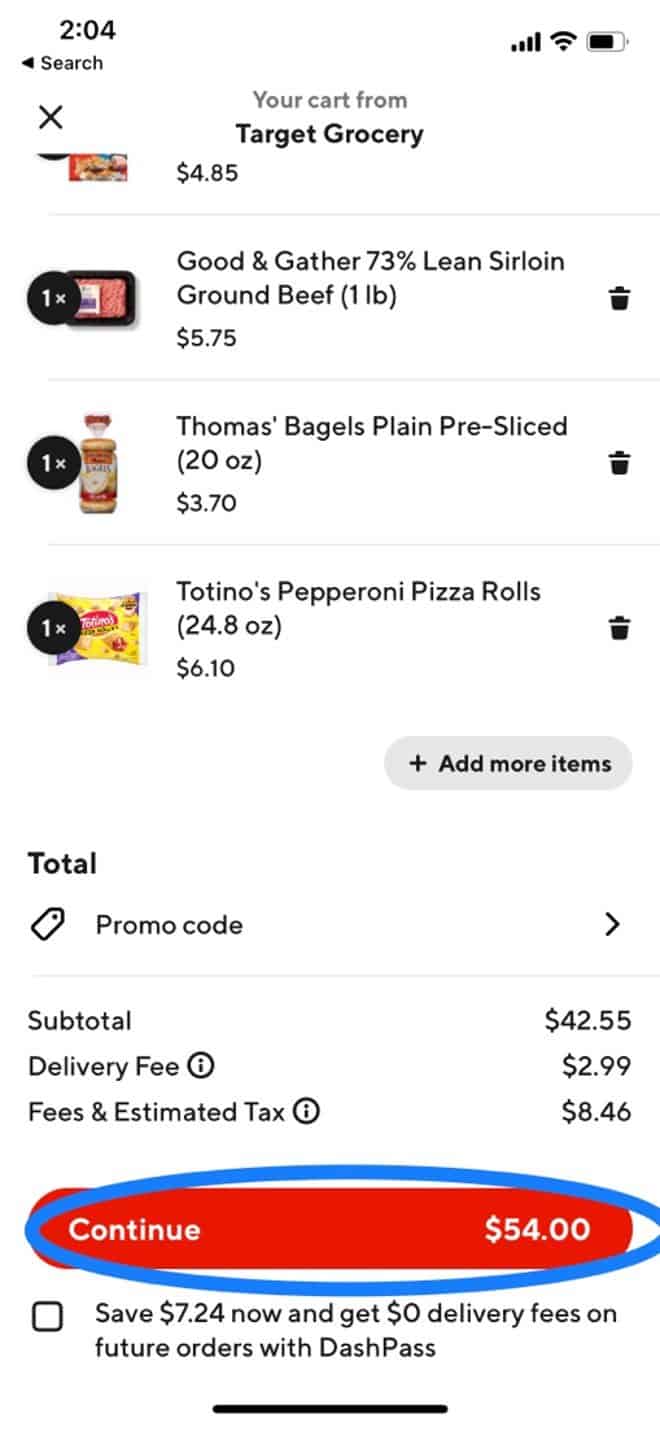This is a detailed description of a screenshot taken from a mobile device displaying a Target grocery shopping cart. 

At the top of the screen, on the left-hand corner, it reads "2:04 PM," and on the right-hand corner, there are indicators for phone signal strength, Wi-Fi connectivity, and battery status. 

Below that, the "Good & Gather 73 Lean Sir" item is prominently featured with a picture of the item against a black circular background, and a white "1x" icon indicating the quantity. Directly below this, the price is listed as $5.90-$7.50, with a trash can icon nearby for deletion.

Following that, additional items are listed:
- "Thomas Bagels (Pre-Sliced)" priced at $3.70
- "Totino's Pepperoni Pizza Rolls" priced at $6.10

There is an option to add more items using a plus (+) button. The subtotal for the items is displayed as $42.55, with a delivery fee of $2.99 and estimated tax and fees totaling $8.46, bringing the overall total to $54.00.

An icon is present for entering a coupon or promo code. The option to proceed to checkout is highlighted in red, with the total cost ($54.00) prominently displayed in blue with a circular background. Near the bottom, there is a checkbox option labeled "Save."